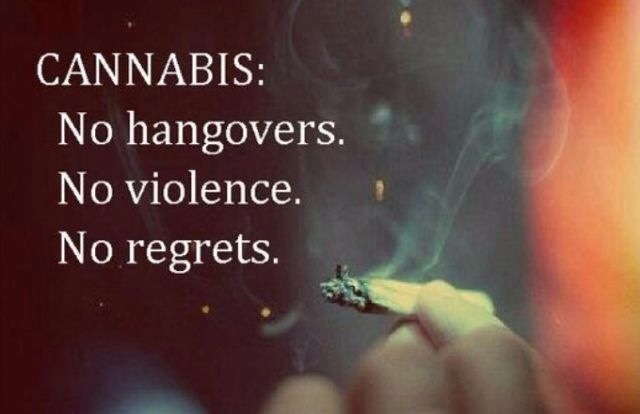The image portrays a promotional sign featuring a detailed illustration on a primarily dark background with a touch of orange light on the right side. The focal point of the sign is a hand, prominently displayed on the right, holding a nearly finished and burning marijuana joint with smoke visibly rising from it. The left side of the image is dominated by bold, white text written in all capital letters, organized into four stacked lines: "CANNABIS," followed by "No hangovers," "No violence," and "No regrets," each punctuated with a period. The sign is presumably created by a special interest group aiming to promote cannabis for advertising or legal advocacy purposes, emphasizing the purported benefits of cannabis use over other substances.